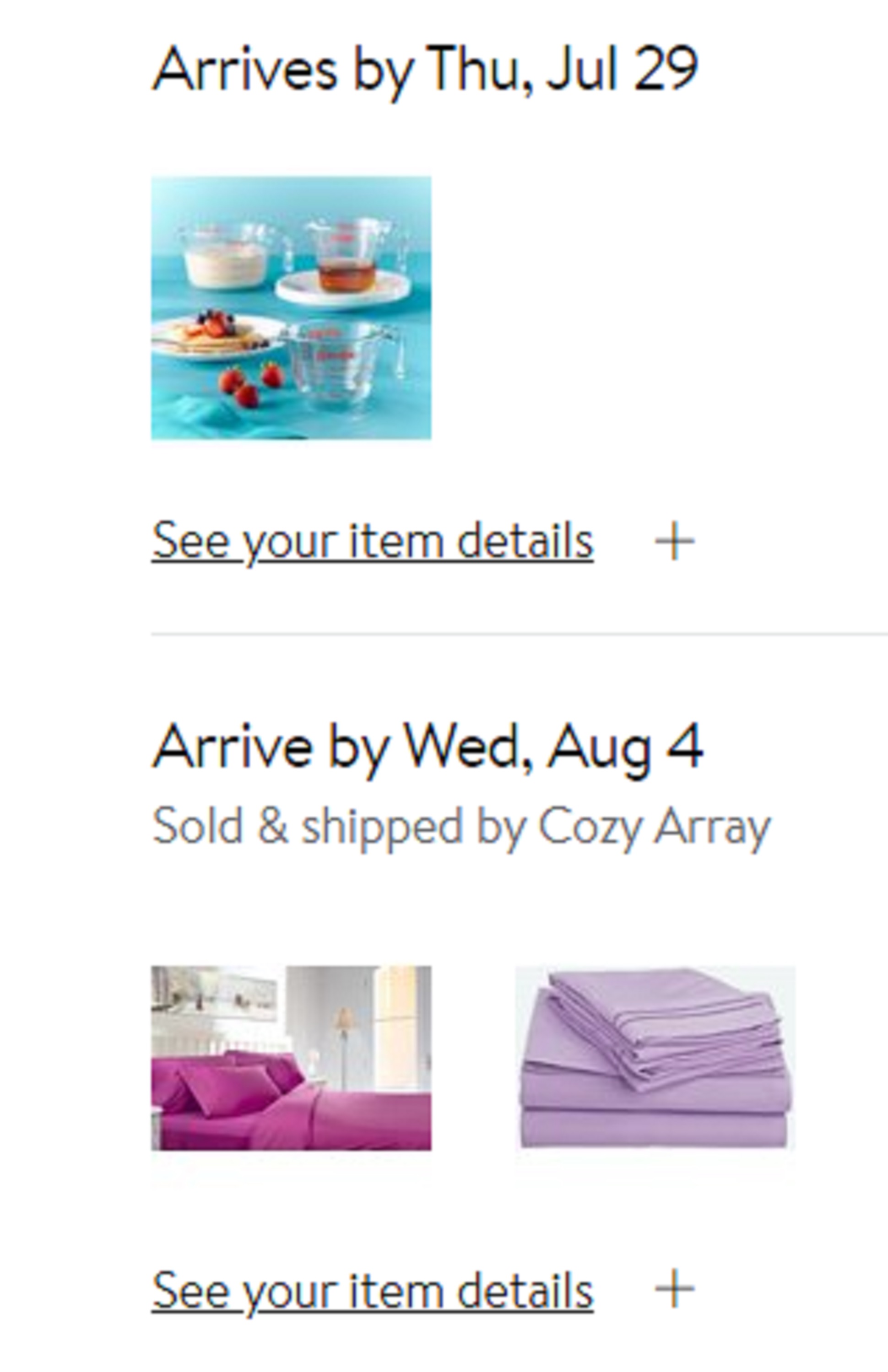A detailed caption for the image could be:

"In the foreground, a trio of clear glass Pyrex measuring cups is meticulously displayed on a vibrant turquoise surface. The ensemble comprises one large and two medium-sized cups, with one cup filled with a rich amber liquid, possibly syrup, and another containing a milky white liquid. Accompanying the measuring cups is a white plate stacked with tan-colored pancakes, garnished generously with red strawberries and blueberries, adding a colorful contrast to the scene.

Above this arrangement, text on a clean white background indicates the expected delivery dates: 'Arrives Thursday, July 29th' for the Pyrex measuring cups. A gray line beneath this section reads 'Arrived by Wednesday, August 4th,' denoting the delivery information for another product sold by and shipped by Cozy Array.

Further detailing below, the image shows two sets of bed sheets. One set is neatly made on a bed in a soft pink hue, while another set, in a rich purple color, is stacked and folded nearby. Both sets are accompanied by the text 'See your item detail,' underlined with a plus sign, indicating additional information available. This comprehensive scene captures an online purchase confirmation displaying both kitchenware and bedding items, complete with their respective delivery schedules."